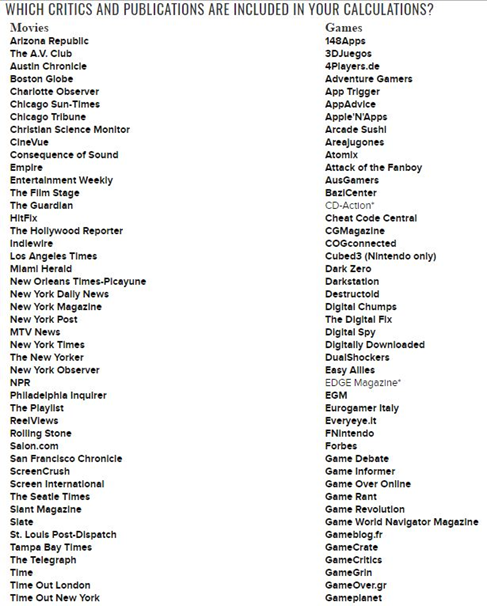In this image, which appears to be a graphical representation of a compiled list, we see two distinct columns of text. On the left side, there is a detailed alphabetical list of movie critics and publications, while on the right side, there is a corresponding list of games.

The text itself is organized in a vertical manner, and each entry is clearly delineated. At the very top of the image, a light grayish colored text provides a context for the list, asking the question, "Which critics and publications are included in your calculations?"

Focusing on the left side, the movie critics and publications are as follows, in alphabetical order: 

- Arizona Republic
- The A.V. Club
- Austin Chronicle
- Boston Globe
- Charlotte Observer
- Chicago Sun-Times
- Chicago Tribune
- Christian Science Monitor
- Cineview
- Consequence of Sound
- Empire
- Entertainment Weekly
- The Film Stage
- The Guardian
- HitFix
- The Hollywood Reporter
- IndieWire
- Los Angeles Times
- Miami Herald
- New Orleans Times
- Picon
- New York Daily News
- New York Magazine
- New York Post
- MTV News
- New York Times
- The New Yorker
- New York Observer
- NPR
- Philadelphia Inquirer
- The Playlist
- ReelViews
- Rolling Stone
- Saloon.com
- San Francisco Chronicle
- Screen Crush
- Screen International
- The Seattle Times
- Saint Magazine
- Slate
- St. Louis Post-Dispatch
- Tampa Bay Times
- The Telegraph
- Time
- Time Out London
- Time Out New York

This comprehensive list aligns precisely from top to bottom, maintaining a logical and easy-to-read format for quick reference.